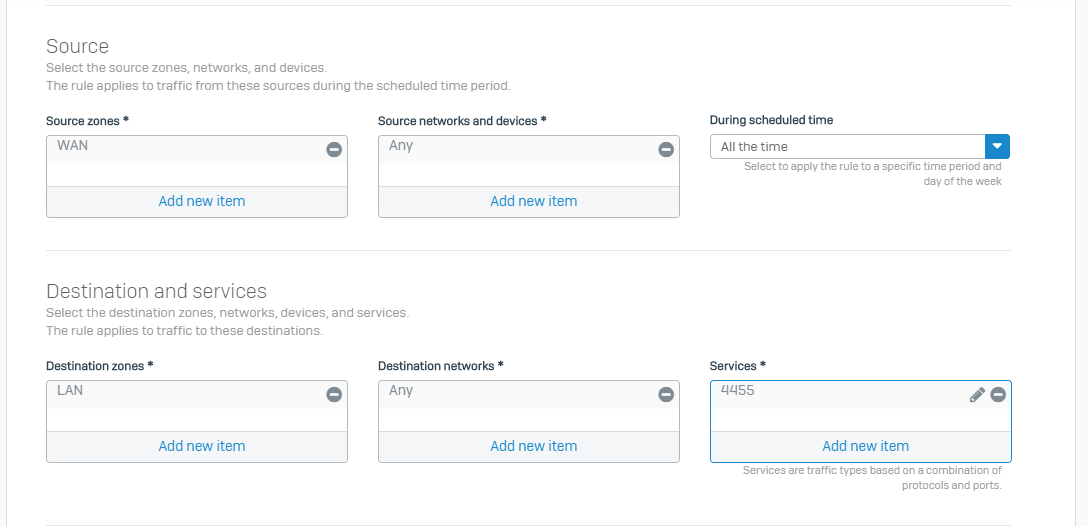This is a detailed screenshot from an application interface of unknown origin, predominantly consisting of text and form fields related to network configuration. At the top, the header reads: "Source. Select Source Zones, Networks, and Devices. The rule applies to traffic from these sources during the scheduled time period." Below, under "Source Zones,” the entry "WAN" is listed with an option to "Add New Item." Similarly, under "Source Networks and Devices," the entry "NE" is available with an "Add New Item" option. The scheduled time period is set to "All the Time," and users can select this to apply the rule to a specific time period and day of the week.

Further down, the section "Destination and Services" instructs users to select the destination zones, networks, devices, and services the rule will apply to. In "Destination Zones," the entry "LAN" is listed with "Add New Item" available. Similarly, "Destination Networks" includes "NE" with an "Add New Item" option. For "Services," the entry "4455" is visible along with a pencil icon, implying an option to edit, and an "Add New Item." It is noted that services refer to traffic types based on a combination of protocols and ports.

The image is formatted in a landscape orientation, being wider than it is tall, and entirely devoid of any living entities or architectural elements. It contains no people, animals, plants, flowers, trees, buildings, automobiles, motorcycles, or airplanes. The content is strictly technical, focusing on network and traffic rules configuration.